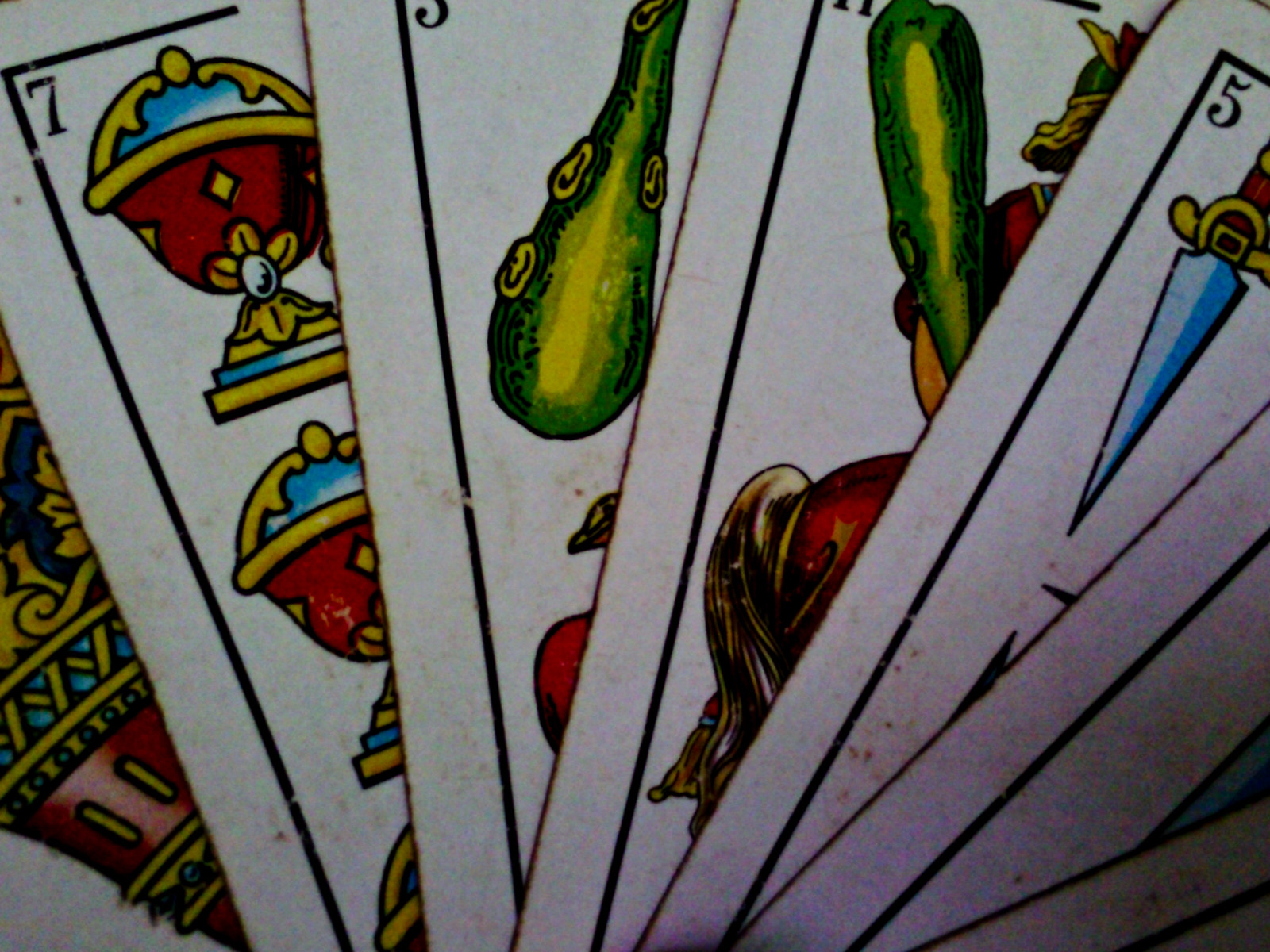The image is a close-up, rectangular photograph featuring a fan arrangement of seven playing cards or tarot cards, layered and overlapping. The overall orientation of the image shows that the top and bottom sides are longer than the left and right. 

At the far left, the bottom-most card displays a single chalice or cup adorned in intricate red, gold, and blue patterns against a white background. Stacked directly above it, the next card features a black border with the numeral "7" in the top left corner and depicts several round, red cups accented with gold details. 

Further up, another card with a black border and white background bears the number "3" in the top left corner. This card partially shows a green club or vegetable as well as a segment of a red apple, obscured by the card above it. 

The fourth visible card, which also has a black border and an out-of-frame number in the top left corner, displays a person gripping a green club. Additionally, the person appears to be mounted on a horse, with the horse's back partially visible.